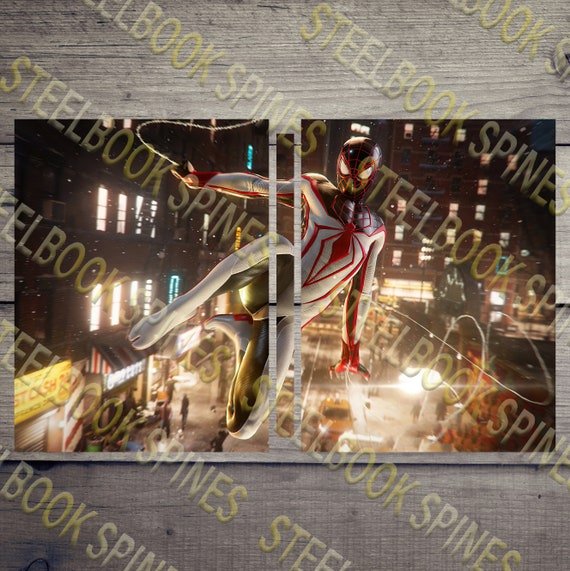The image features a photograph of a weathered wood background, primarily gray, that frames the entire scene from the top, bottom, and a narrow strip along the sides. Superimposed on this background is a vibrant, dynamic poster of Spider-Man swinging through an urban landscape at night. The Spider-Man in this image dons a unique suit, predominantly white with striking red markings. A large red spider emblem dominates his chest, with spider legs extending down his arms. His mask is red and black with shining eyes, adding an intense visual element. Notably, his feet feature a distinct design, with the big toes separated from the rest, resembling a hoof. The background captures a well-lit cityscape, complete with high-rise buildings and a shopping district below, where a bustling market and numerous lit windows can be observed. Throughout the entire image, a light yellow watermark repeatedly reads "Steelbook Spines" in multiple rows from the top left to the bottom right, slightly obscuring the view, yet allowing the vivid details of Spider-Man and the city to remain prominent.